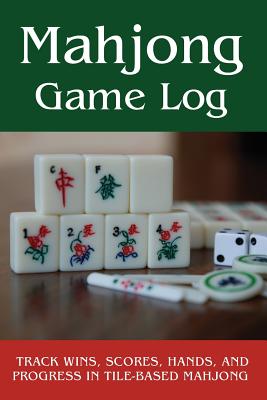The image features the cover of a Mahjong game log book. At the top, white letters on a dark green background spell out "Mahjong Game Log." Below this, taking up the middle third to half of the image, is a photograph of Mahjong tiles, dice, and other game accessories arranged on a polished wooden tabletop. The tiles showcase a variety of designs, including floral patterns and Chinese characters, with numbers ranging from one to seven. Notably, some tiles display a red 'C' and a green 'F.' The dice are white with black dots; one prominently shows two dots while another, partly visible, shows one dot. Additionally, there are circular coins encircled in green with blue designs and white, stick-like objects bearing similar floral motifs. At the bottom, a red banner with white text reads, "Track wins, scores, hands, and progress in tile-based Mahjong." The photograph and text layout suggest that this is either a book cover, an advertisement, or the top of a game box.